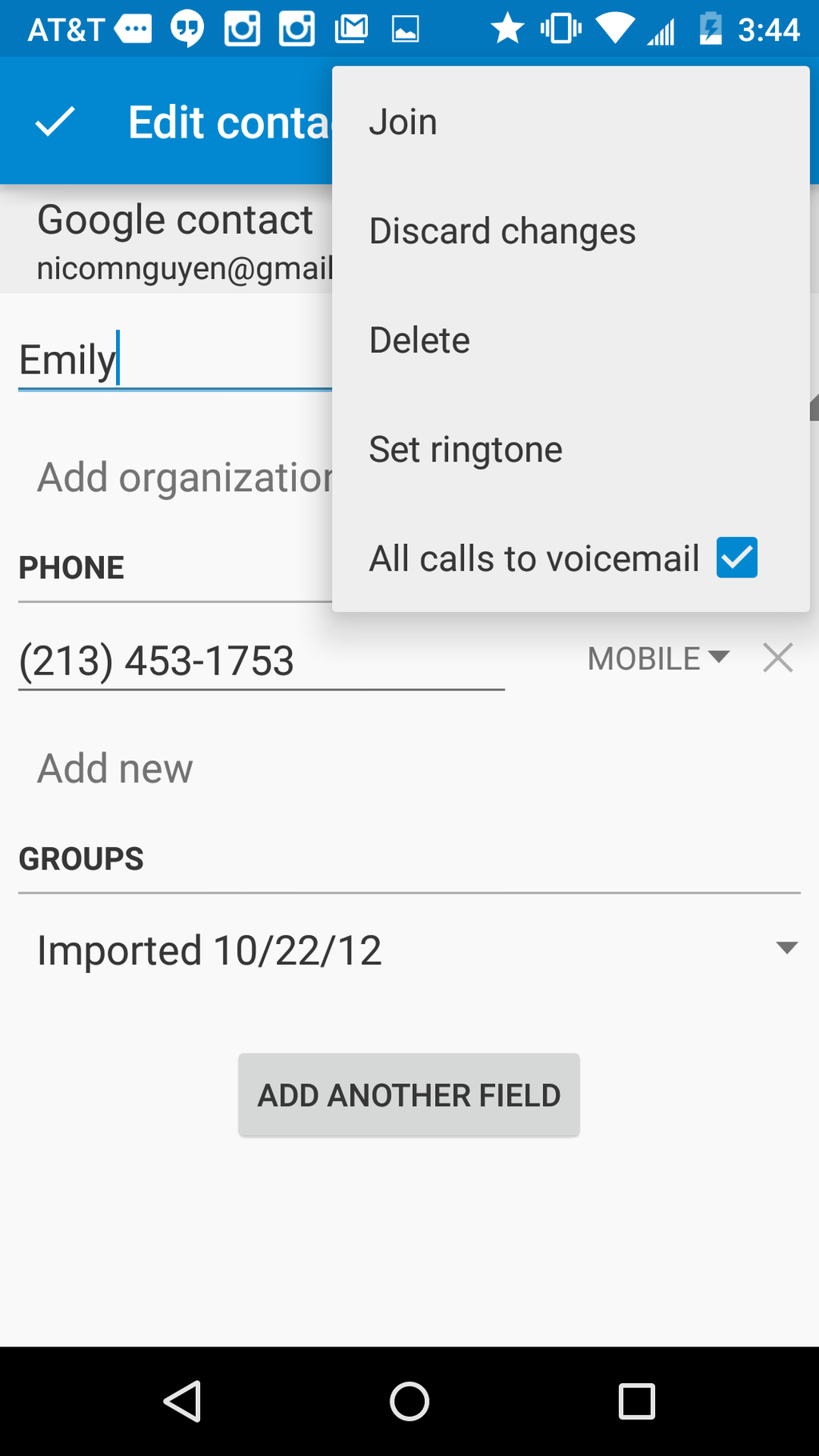The image shows an Android phone screen with the contact editing interface open. The contact name entered is "Emily Nguyen," with the specific spelling "N-G-U-Y-E-N-D-A" for the last name. An email address is visible, which is a Gmail account, though it’s unclear if it belongs to Emily or the phone owner. The phone number listed has a 213 area code. The "organization" field appears blank, and there is a note saying the contact was imported on October 22, 2012. Additional options are selected, including "join," "discard changes," "delete," "set ringtone," or "all calls to voicemail." The latter option is checked, indicating that any calls from Emily will go straight to voicemail. There's a check button in the top left corner to save the changes, and an "add another field" button for adding more information to the contact.